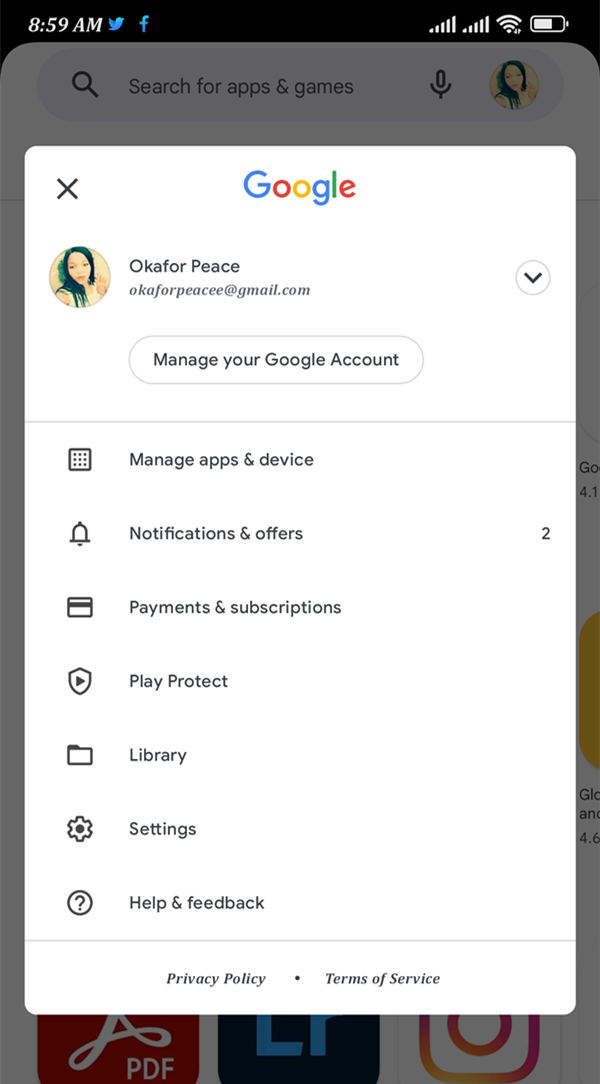The screenshot displays a user's mobile interface at 8:59 a.m. In the upper left corner, there's the time alongside the blue Twitter bird icon, followed by the lowercase "f" for Facebook, indicating sharing options. To the right, the battery icon shows near full charge, and the signal strength displays five bars.

Below this, a long vertical box starts with an 'X' in the upper left corner. To its right, the "Google" logo is positioned next to a small circular profile picture. The profile picture depicts a young woman in her early 20s, with long black hair, red lips, and brown eyes. Below the image is the name "Okafor Pease," followed by her email address: "okaforpease@gmail.com".

Below her email, within a long horizontal bar, is the option to "Manage your Google Account". Subsequent subcategories include "Manage apps and device" (icon of a bell), "Notifications and offers" (credit card icon representing payments and subscriptions), "Play Protect", "Library", and "Settings". Finally, there's a circular icon with a question mark labeled "Help and feedback".